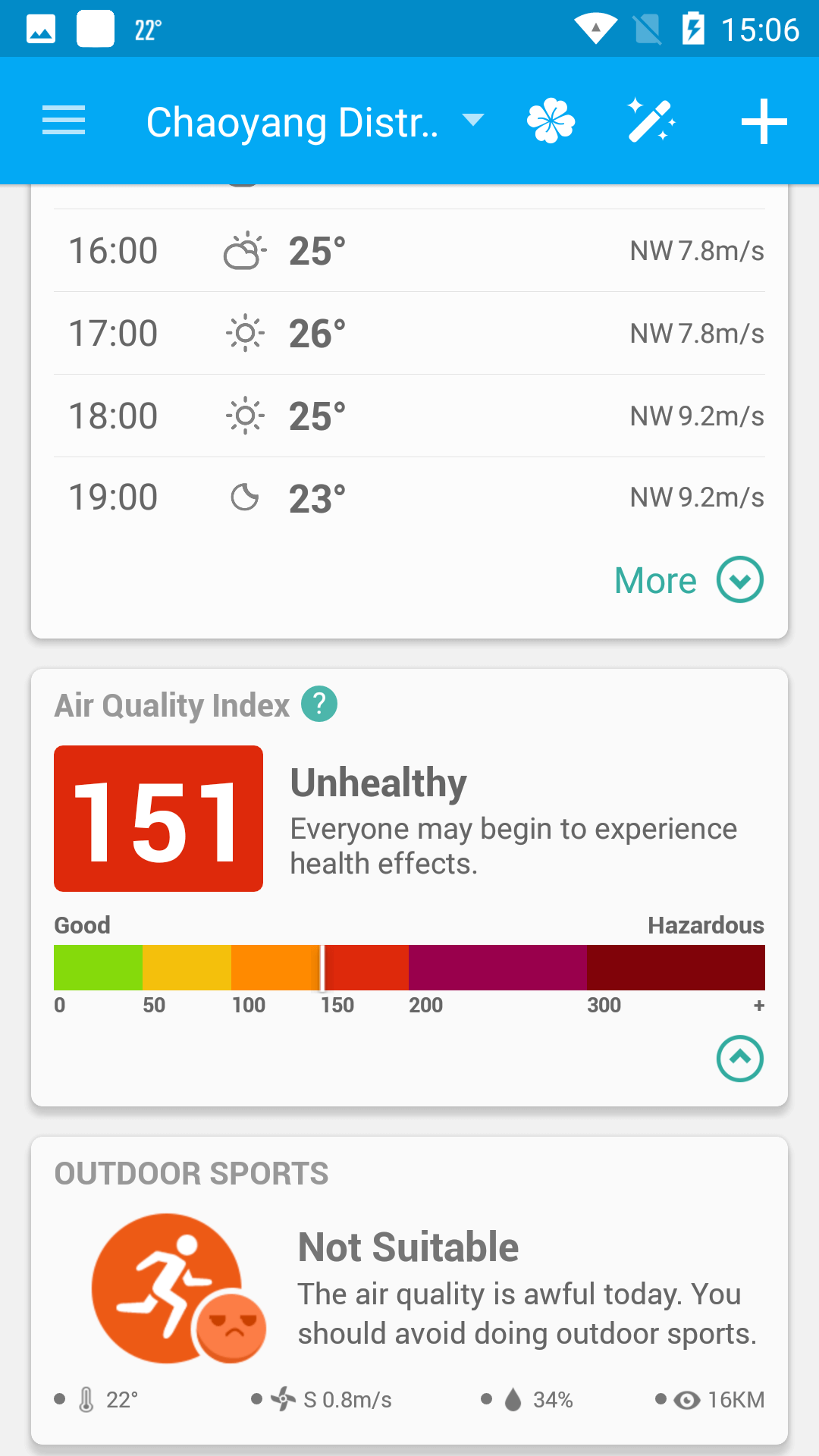**Detailed Weather and Air Quality Update for Chaoyang District**

*Weather Overview:*
- **Location:** Chaoyang District
- **Change Location Option:** Available via a dropdown box
- **Icons Present:** Shamrock, magic pen, and plus symbol

*Current Time and Status:*
- **Taskbar Time:** 15:06
- **Battery Status:** Charging (indicated by a lightning bolt)
- **Wi-Fi:** Connected
- **Temperature:** 22°C
- **Conditions:** Partly to mostly sunny
- **Wind:** Northwest at 8 mph

*Weather Timeline:*
- **16:00:** 25°C, partly to mostly sunny
- **17:00:** 26°C, sunny
- **18:00:** 25°C, sunny
- **19:00:** 23°C, dark

*Air Quality Information:*
- **Current AQI:** 151 (Unhealthy) - Red Box
- **Health Advisory:** "Everybody may begin to experience health effects."
- **AQI Scale:** From 0 (Good/Green) to 300+ (Hazardous)

*Outdoor Activity Recommendation:*
- **Sports Suitability:** Not suitable
- **Advisory:** "Awful today. You should avoid doing these sports."
- **Visual Indicator:** Runner icon with a sad emoji